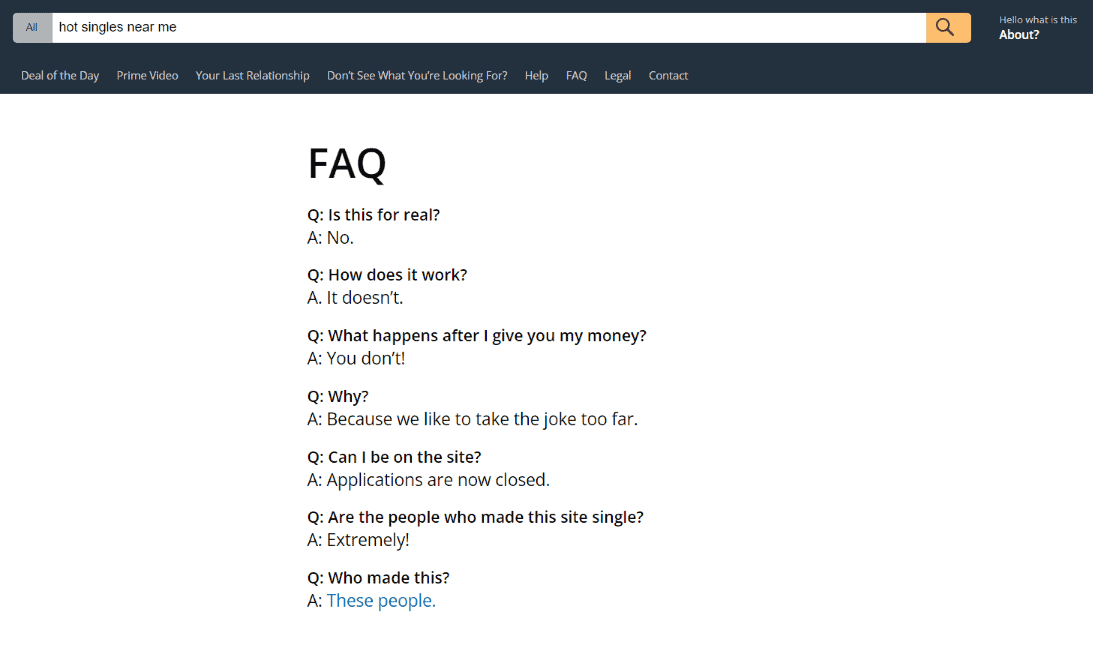This screenshot captures a humorous and spoofed Amazon Prime page. At the top, there's a search bar containing the amusing query "hot singles near me." 

Below the search bar, there are several navigation options including "Deal of the Day," "Prime Video," "Your Last Relationship," "Don't See What You're Looking For?," "Help," "Frequently Asked Questions," "Legal," and "Contact."

The main section of the screenshot prominently displays a "Frequently Asked Questions" section featuring a series of tongue-in-cheek Q&A:

1. **Question**: Is this for real? 
   **Answer**: No.
2. **Question**: How does it work? 
   **Answer**: It doesn't.
3. **Question**: What happens after I give you money? 
   **Answer**: You don't.
4. **Question**: Why? 
   **Answer**: Because we like to take the joke too far.
5. **Question**: Can I be on the site? 
   **Answer**: Applications are now closed.
6. **Question**: Are the people who made this site single?
   **Answer**: Extremely.
7. **Question**: Who made this? 
   **Answer**: These people.

The background of the screenshot is predominantly white, contributing to the clean and minimalist look of the page.